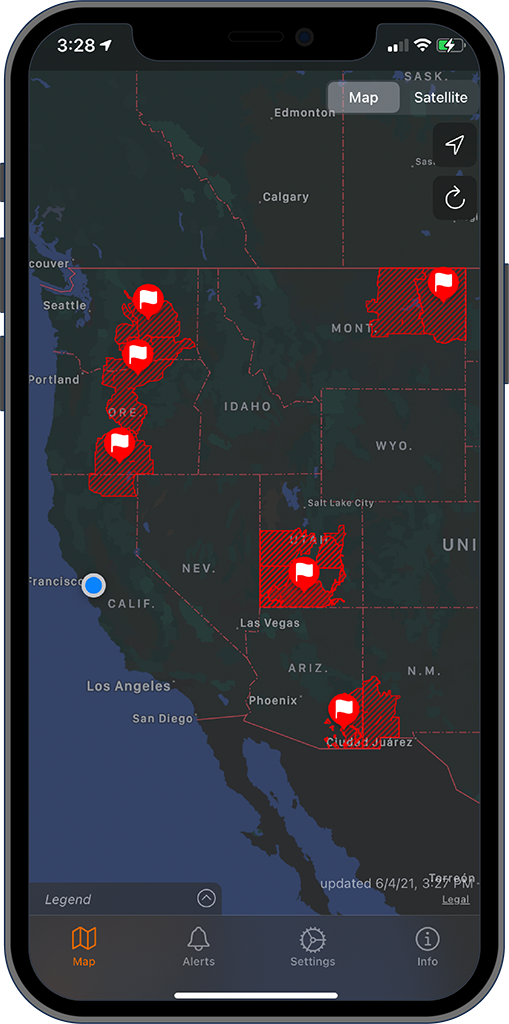In this screenshot of a black cell phone screen, the time displayed in the upper left corner reads 3:28. The screen shows a map of the western United States, covering areas from Wyoming and Montana down to New Mexico and westward. The map is depicted in black with mountain regions shaded in forest green. Prominent cities such as Seattle, Portland, San Francisco, Los Angeles, and San Diego are labeled in white text. A region is marked prominently in red, outlined with six white flags, indicating specific locations: one in Arizona, one in Montana, and three in Oregon.